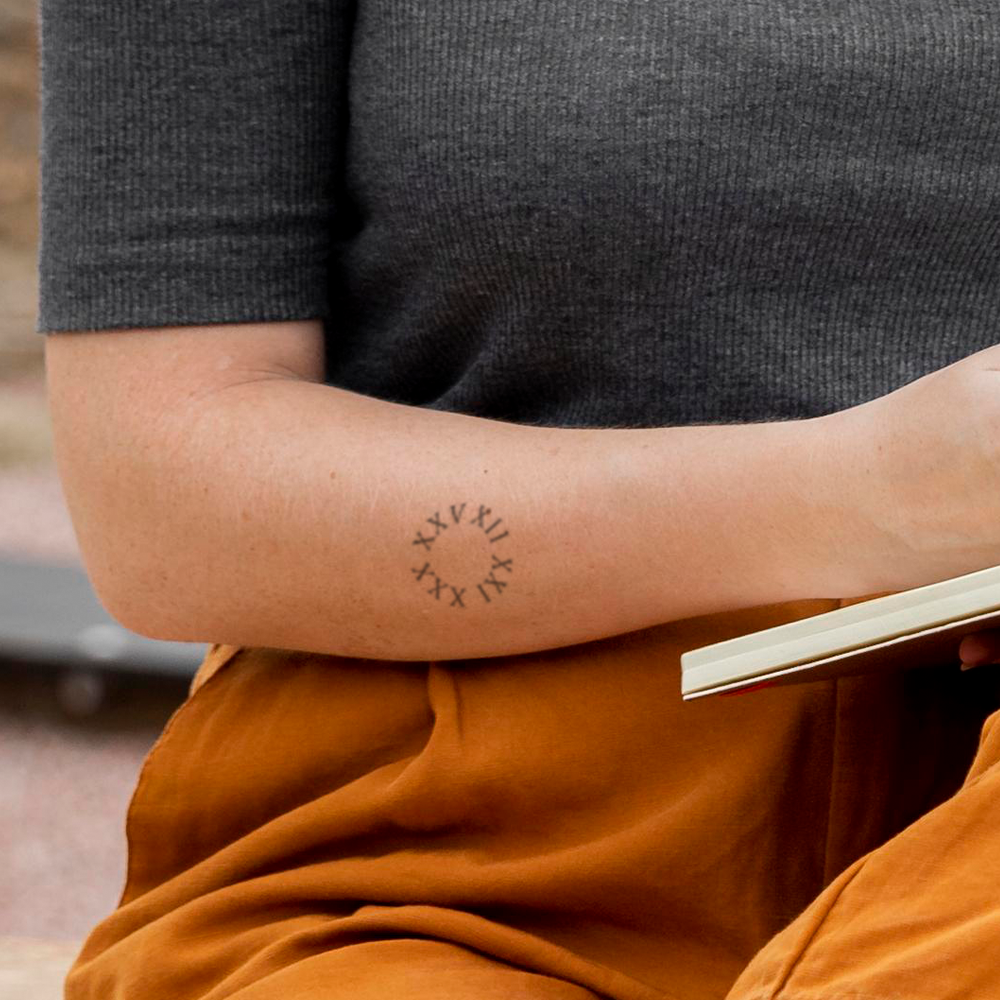The photograph captures the lower chest to upper thigh portion of a seated Caucasian individual, suggesting an outdoor setting with a bright, blurred background. They are dressed in a gray, slightly form-fitted top, with sleeves ending just above the elbows, and orange bottoms featuring a ruffled waist. The individual's arm prominently displays a circular arrangement of Roman numerals: XXV, XII, XXI, XXX, and XXV. They are holding an open book, with no other legible text visible in the image.